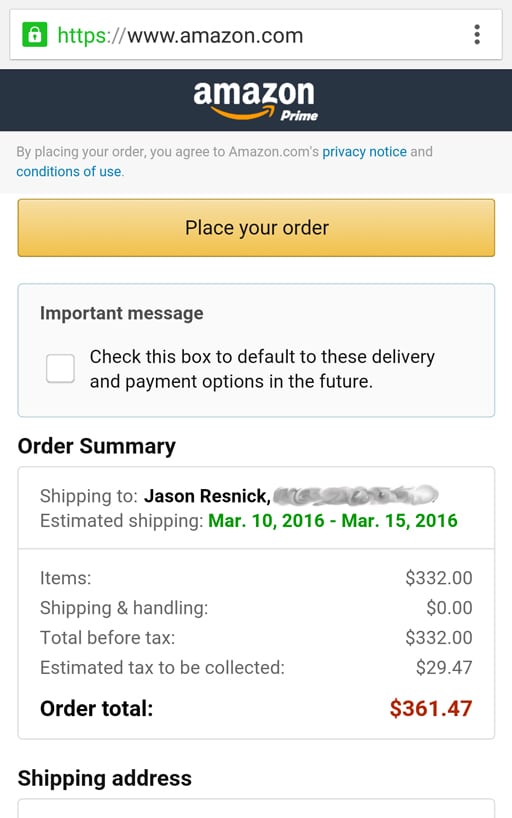The image is a screenshot of an Amazon order confirmation page displayed on a mobile device in portrait orientation. At the top of the screen, there's a secure search bar with a green padlock icon, indicating HTTPS encryption, followed by the URL "www.amazon.com". Directly below it, a black bar stretches across the screen with "Amazon Prime" written in white letters.

Further down, there is a disclaimer in small gray text that states, "By placing your order, you agree to Amazon's privacy notice and conditions of use," with "privacy notice" and "conditions of use" highlighted in blue, indicating clickable links. Below this, a prominent, orange, rectangular button labeled "Place your order" is centrally displayed.

Underneath the button, there's a blank white space followed by a pale gray-outlined rectangle containing the text "Important message." This section has a checkbox with the instruction, "Check this box to default to these delivery and payment options in the future."

Following this, "ORDER SUMMARY" is written in all caps, indicating a breakdown of the purchase details. The first section displays "Shipping to: Jason Resnick" in bold letters, with some information to the right obscured. The estimated shipping date range is shown in green text as "MAR 10, 2016 to MAR 15, 2016".

The cost breakdown follows: 
- Items: $332.00
- Shipping and Handling: $0.00
- Total before tax: $332.00
- Estimated tax to be collected: $29.47

The order total, highlighted in bold red, is $361.47.

Lastly, the screenshot cuts off at the "Shipping address" section, leaving the rest of the screen unseen.